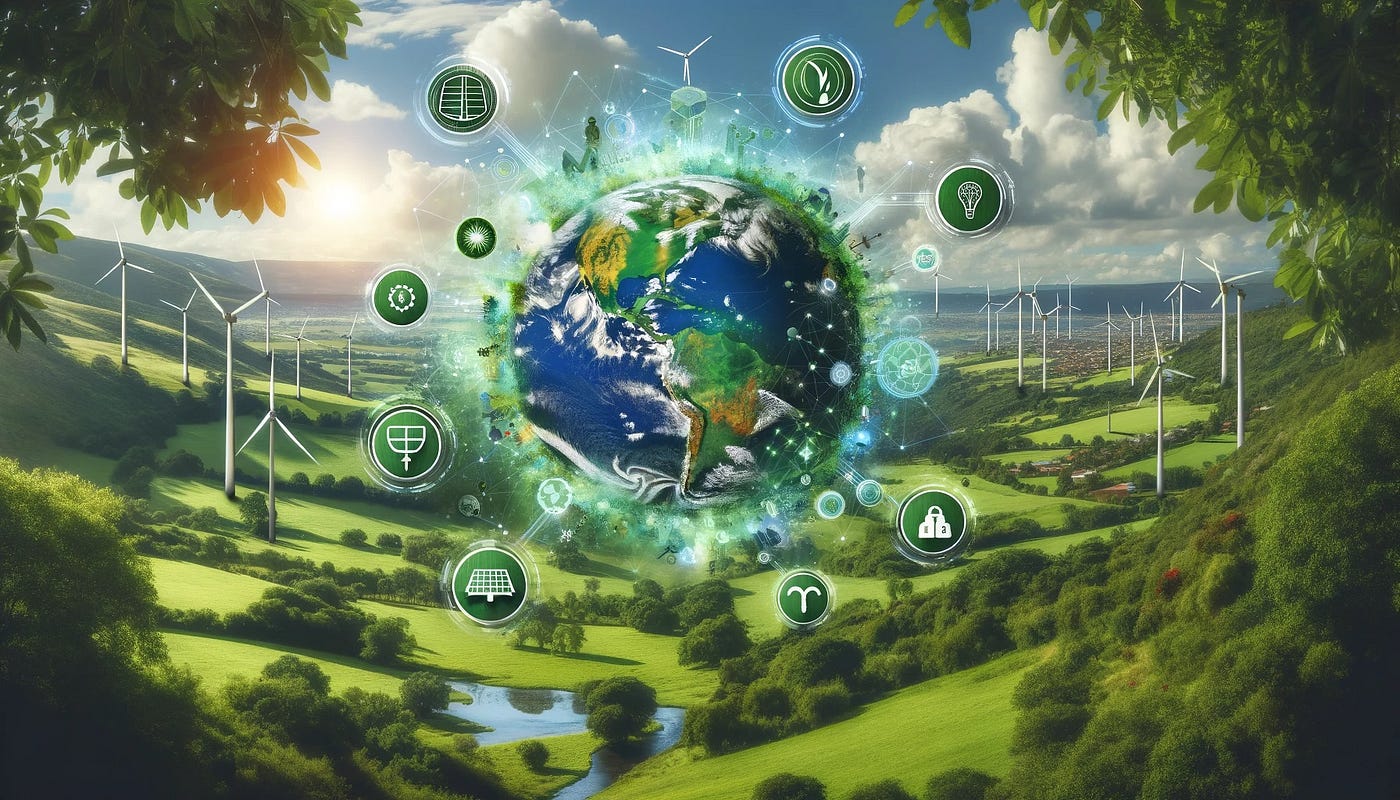The image is a computer-generated or AI-generated art piece showcasing a vibrant and detailed landscape. In the foreground, there are close-up leaves from trees framing the sides and top corners of the image. The scene features rolling hills adorned with scattered trees, serene lakes, and wind turbines dotting the farmland, indicative of a wind farm. The farmland is characterized by deep green, manicured grass with surrounding forests.

Dominating the center of the image is a digitally stylized planet Earth, prominently highlighting North and South America. This globe emits a glowing green and white aura. Encircling the Earth are various green circles with white icons inside, resembling modern digital buttons or symbols, with eight or nine larger circles and several smaller, almost transparent light blue ones.

In the background, a clear blue sky with puffy white clouds and a yellow sun extends over the landscape, providing a serene and hopeful ambiance. The overall composition conveys themes of environmental preservation and sustainable energy through the depicted wind farms and digital symbols around the glowing Earth.